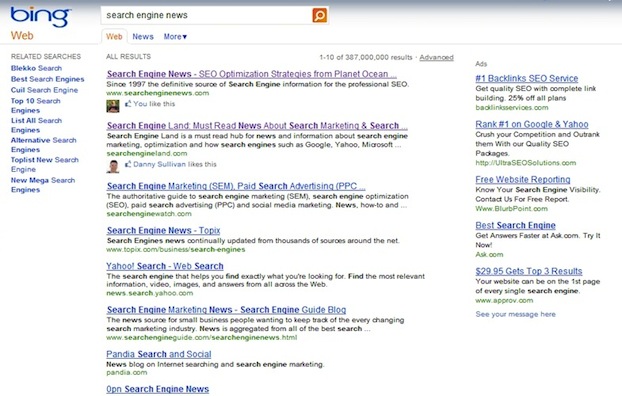The image depicts Bing search results for "Search Engine News." On the left-hand side, a section titled "Related Searches" lists the following queries: "BLECO Search," "Best Search Engines," "KUIL," "Cuil Search Engine," "Top 10 Search Engines," "List All Search Engines," "Alternative Search Engines," "Topless New Search Engine," and "New Mega Search Engines." 

On the right-hand side, there are various advertisements, though specific details are not provided.

The main search results in the center show that two links have already been visited, highlighted in purple. The first clicked-on link is for "Search Engine News," which provides information on SEO Optimization Strategies from Planet Ocean and is the definitive source of search engine information for professional SEOs since 1997. The URL is www.searchenginenews.com, and it shows a Facebook "Like" icon to denote user approval.

The second clicked-on link is for "Search Engine Land," described as a must-read hub for news and information about search engine marketing, optimization, and how search engines like Google, Yahoo, and Microsoft function. The URL features an endorsement from Danny Sullivan, a notable figure in the field.

Other search results are listed but have not yet been clicked on, offering additional resources and articles related to search engine news.